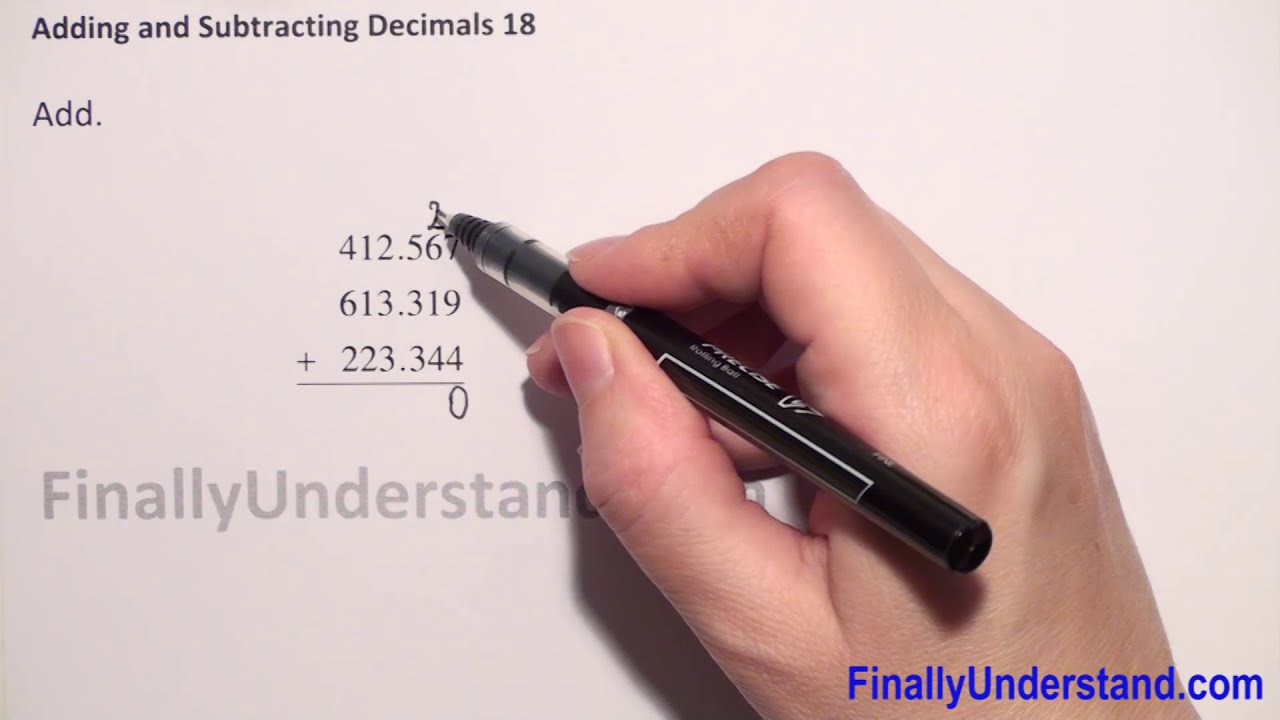The image features the title "Adding and Subtracting Decimals 18" prominently displayed in the top-left corner on a gray background. Below this title, the word "Add" is written, followed by an arithmetic equation. The equation includes the numbers 412.5627, 113.319, and 223.3440, with these values stacking vertically as an addition problem. A human hand, positioned on the right side of the image, holds a black marker and begins solving the problem by writing a zero under the four and carrying a two above the six. The hand appears to be in the process of demonstrating the addition method. At the bottom right corner of the image, the URL "finallyunderstand.com" is visible, suggesting that the image may be part of an educational resource or a live stream explaining how to perform decimal additions. The image has a bright, educational aesthetic with colors like white, black, and blue, giving it a clean, instructional appearance.